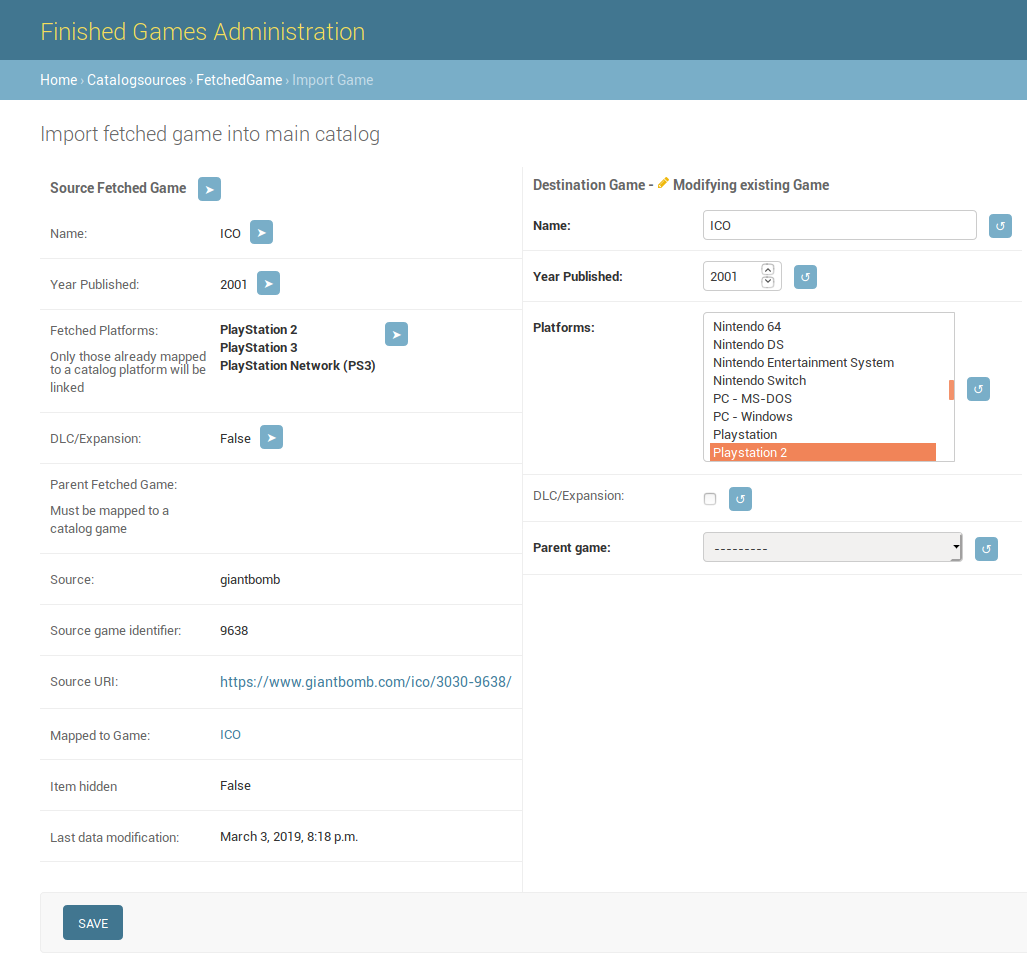This image displays a detailed user interface for managing and importing games into a catalog. At the top, the interface is identified as "Finished Games Administration" and includes multiple sections labeled as "Home," "Catalog," "Source," and "Fetched Games." Below this, there's an option to "Import Fetched Games into Main Catalog."

Further down, the interface details some specific attributes for a game named "ICO." The game's publish year is marked as 2001, and it is available on several platforms: Playstation 2, Playstation 3, and Playstation Network (PSN) for PS3. The note specifies that only platforms already mapped in the catalog will be linked. 

Additional information includes:
- DLC/Expansion status: False
- Parent Fetched Game: Not specified, must be mapped to a catalog game
- Source: Giant Bomb
- Source Game Identifier: 9638
- Source URI: https://www.giantbomb.com/ICO/3030-9638/
- Map to Game: "ICO"
- Hidden Item Status: False
- Last Date Modified: March 3, 2019, at 8:18 PM

At the bottom of the interface, there is a teal-colored save button with white font available for the user to confirm and save these settings.